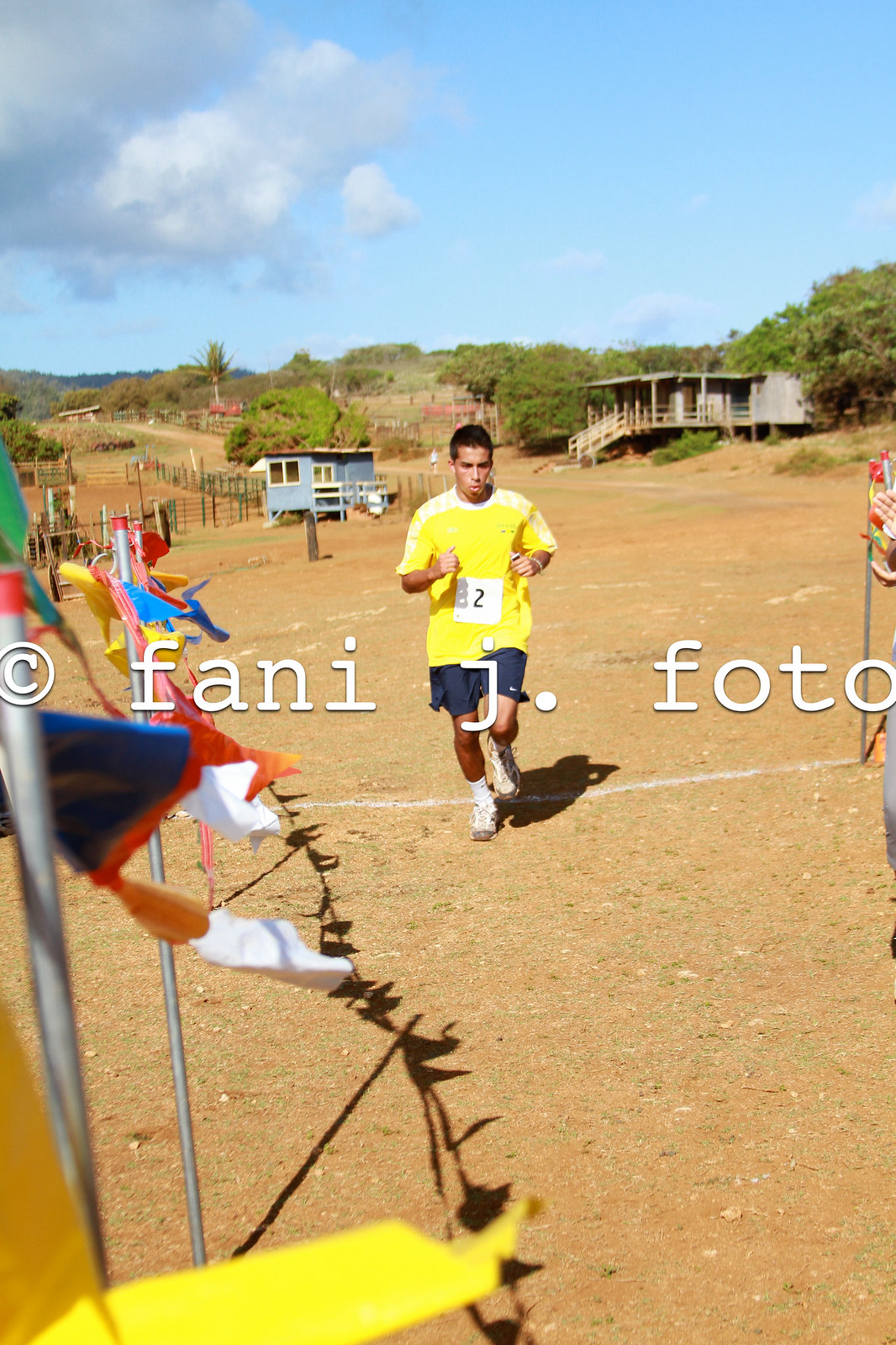In the image, a man with a full head of black hair and relatively dark skin is seen running, possibly nearing the finish line of a marathon or race in a hot, arid location that resembles a desert or sub-Saharan landscape. He is dressed in a long, yellow and somewhat baggy shirt paired with blue shorts and wearing running shoes. A white piece of paper with the number 2 is pinned to the front of his shirt. The ground is entirely dirt, and a line drawn in it likely signifies the finish line. Surrounding him are colorful flags, seemingly arranged to guide runners toward the end of the race. The backdrop features two primitive buildings, one blue and stilted, the other tan, with scattered sub-Saharan trees under a clear blue sky. The top of the picture is marked with the text "copyright Fanny J. Foto". The runner appears to be the only participant in the frame, with no spectators visible.